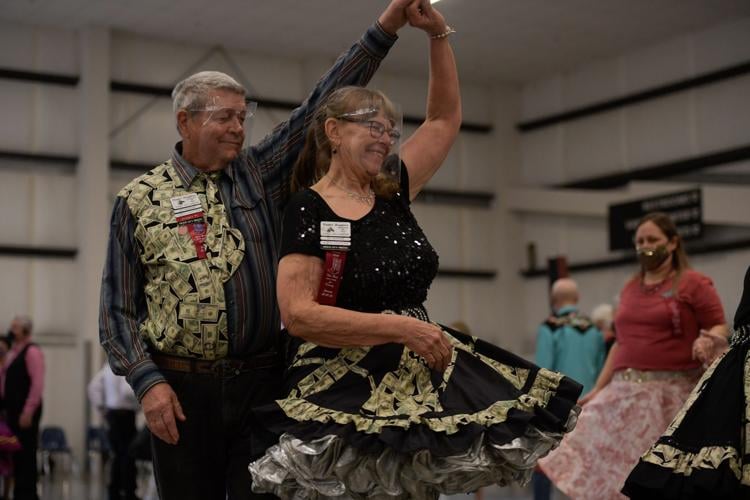The image captures a lively dance performance set outdoors among tall buildings, with natural light brightening the scene. In the foreground, a woman dressed in an elaborate, Mexican-inspired black costume featuring full skirts and petticoats twirls gracefully. She wears a name tag adorned with a red ribbon and clear face mask, her wide smile revealing the joy of the moment. Behind her, an older man also sporting a name tag with a red ribbon and a clear face mask, dressed in a dark gray long-sleeve shirt with ornate decorations and images of money, raises his hand to spin her in a graceful move. The clarity of the photograph highlights the cheerful ambiance, with other mask-wearing onlookers visible in the background, sharing the joyous occasion.